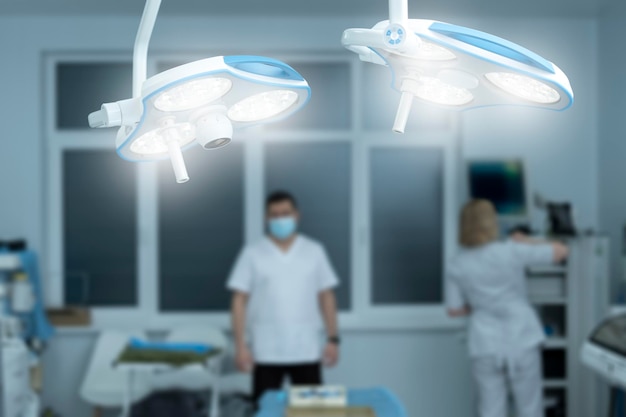The image showcases a scene in a medical facility, likely a doctor's office or an operating room. In the foreground, two triangular-shaped surgical lights hang from the ceiling, each equipped with three bright, circular LED lights arranged in a triangular pattern. The lights are off-white and feature teal handles on both sides, allowing for easy adjustment. These lights are angled to illuminate the area below, suggesting a functional setting.

In the background, against a context of white walls and a window with a white frame, the scene includes two medical staff members. A male nurse wearing a blue mask, a long white shirt, and black pants stands facing the camera. He also has a watch on his wrist. To his left, there is what appears to be a medical tank. Next to him, a female nurse, with her back to the camera, is attending to a screen mounted on a shelf. She is dressed in a typical nurse's outfit, consisting of long white pants and a short shirt. Additionally, there is a hospital bed to the left of the male nurse, enhancing the medical context of the image. Overall, the photograph captures the clinical and professional environment of a healthcare setting, emphasizing the use of advanced lighting equipment and the presence of attentive medical staff.